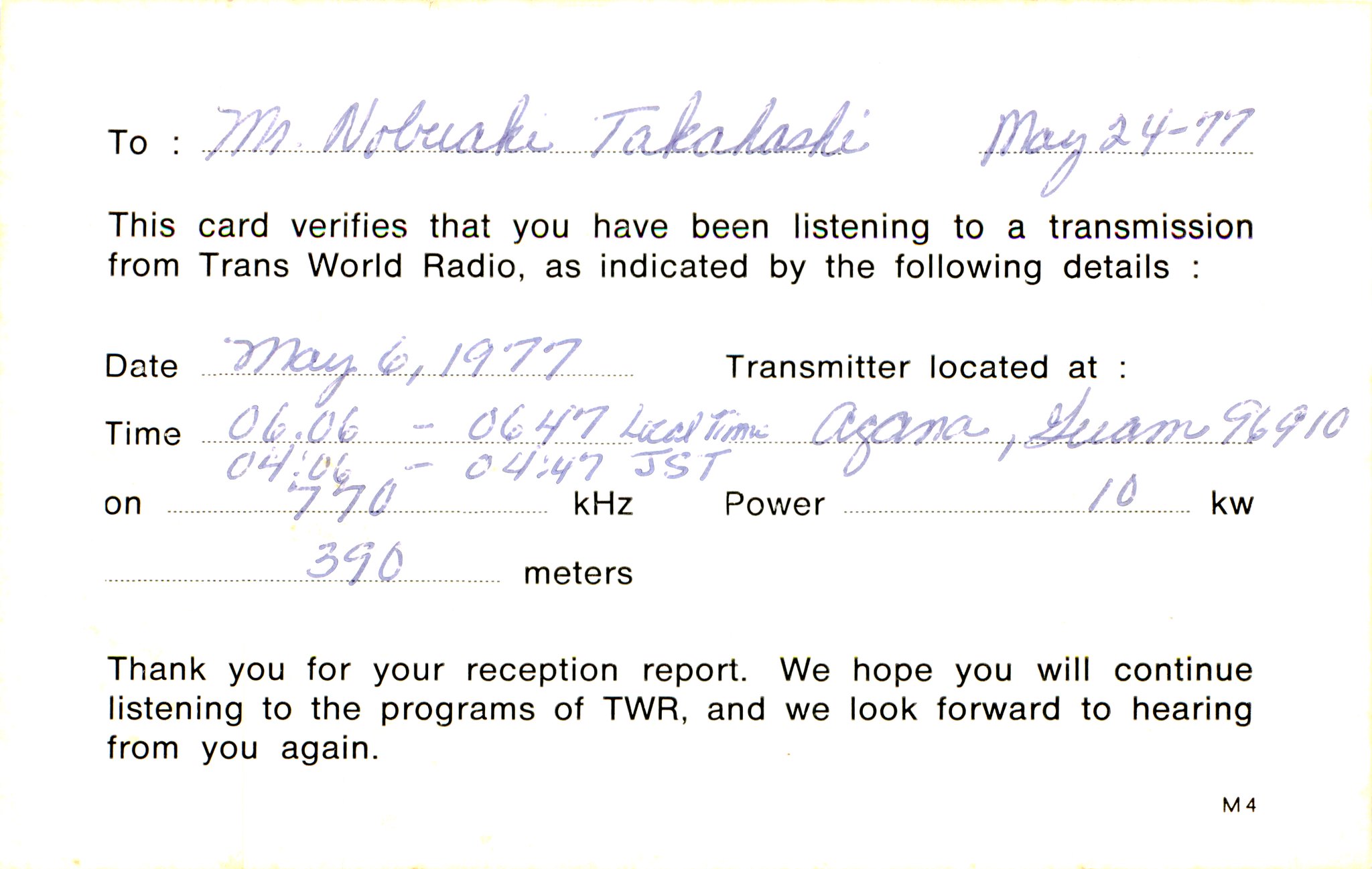The image depicts an old verification card from Trans World Radio, addressed to Mr. Nobaki Takahashi, dated May 27, 1977. The card certifies that Mr. Takahashi was listening to a transmission from Trans World Radio on May 6, 1977. The details of the transmission are meticulously noted: the listening time was from 06:06 to 06:46 local time in Ghana, which corresponds to 04:06 to 04:47 JST on a frequency of 770 kilohertz, with a power of 10 kilowatts, and a wavelength of 390 meters. The card, filled out in blue ink, also includes the illegible transmitter location. The edges of the card are slightly pink against the predominantly white background. The message concludes with a note of gratitude for the reception report, expressing the hope that Mr. Takahashi will continue to enjoy TWR's programs and maintain correspondence.